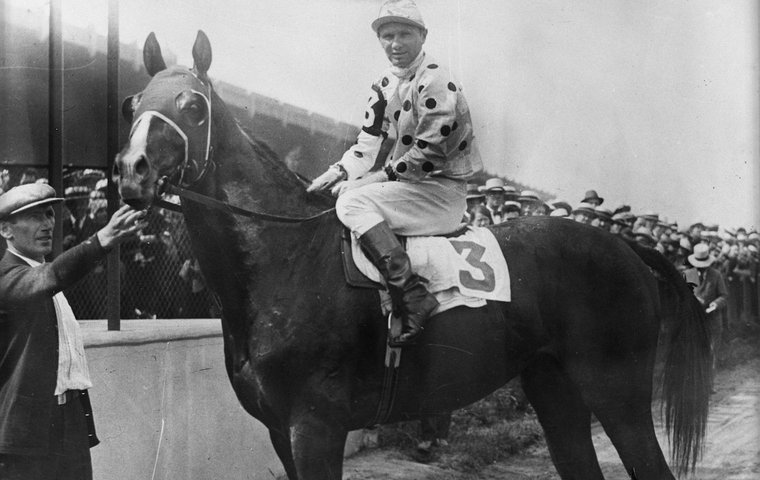This black-and-white photograph appears to be from the 1930s or 1940s, capturing a victorious moment of a jockey and his horse after a race. The jockey is perched atop a beautiful brown horse, which is marked with the number three. The jockey is adorned in a striking polka dot silk shirt, white pants, and tall black boots, completed with a white cap. Facing slightly to the left, he holds the reins while looking towards the front of the image. A man, likely the trainer, stands at the front of the horse, reaching up towards its mouth with one hand. He is dressed in a vintage suit and an old-fashioned hat with a brim, echoing the styles of the early 20th century. In the background, a crowd of predominantly men, all wearing similar hats, watches from the stands and behind a concrete wall. The racetrack appears to be made of dirt, and the sky above looks overcast, lending a nostalgic atmosphere to the scene.